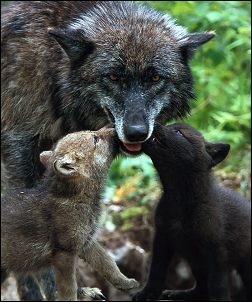This captivating photograph captures a serene moment in nature, featuring a mother wolf and her two cubs nestled in a verdant forest. The image centers around the large, brown-furred mother wolf with shades of white and gray on her face, which is staring directly at the camera, her mouth slightly open. Flanking her are her two adorable cubs, each engaging in a playful display of affection. The lighter-colored cub on the left, with its light brown coat, and the darker cub on the right, almost black with striking blue eyes, both have their mouths touching their mother's, creating a heartwarming scene that resembles a familial kiss. The blurred green foliage in the background, coupled with patches of dirt and possibly rocks, highlights the natural habitat of these majestic creatures. Taken during the daytime, the photograph beautifully captures the tender bond and playful interactions within this wolf family.